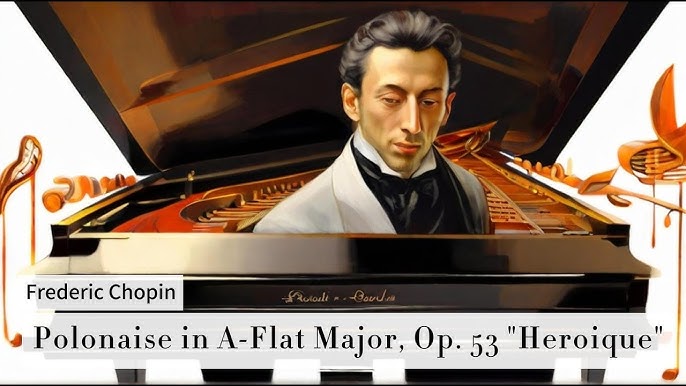The illustration features a stylized, possibly AI-enhanced or hand-drawn depiction of the famous composer Frédéric Chopin. Emerging from an open grand piano with visible strings and hammers, Chopin's upper body dominates the scene. He is portrayed with dark, brushed-back hair and a pensive expression. His attire includes a gray overcoat layered over a black shirt and white shirt. The piano itself is rendered with deep orangish-brown wood and red detailing inside. Text on the image identifies the scene with "Frédéric Chopin" and "Polonaise in A-flat major, Op. 53, 'Heroïque.'" The background is largely white, and various unrecognized decorative elements or instruments flank the piano, adding to the artistic interpretation.